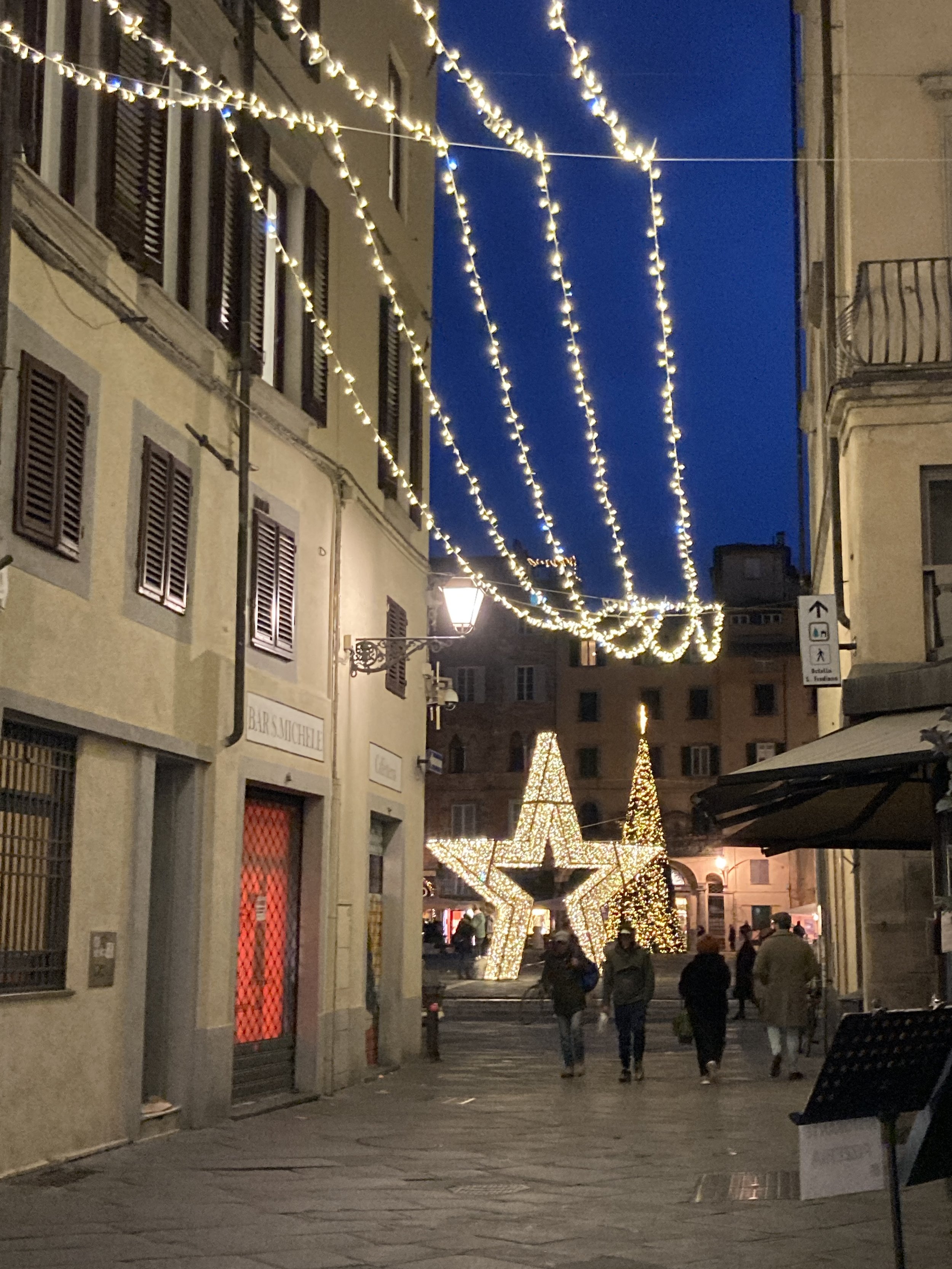This detailed photograph depicts a bustling city street at night, possibly in a small festive district. The scene is set between two tall beige and brown buildings, each featuring a series of windows with closed brown shutters on the lower floors and open shutters on the upper levels. The left building has a brown door with a chain front emanating red light, labeled "Bar S Mitchell," while another similar door on the right emits an orange glow. Festive string lights crisscross the alley from one building to the other. 

A lit street lamp stands at the street's end, adjacent to a support holding it. The dark blue evening sky creates a beautiful backdrop for the festive decorations, including a large lit-up star in the center of the plaza and an even taller illuminated Christmas tree behind it, topped with a distinctive star. Numerous people, dressed warmly in jackets and blue jeans with white shoes, wander through the concrete-lined alleyway. In the distance, we see more individuals near the decorations, enhancing the vibrant and joyous atmosphere of the scene. The right side of the image partly reveals another beige building with railings and windows.